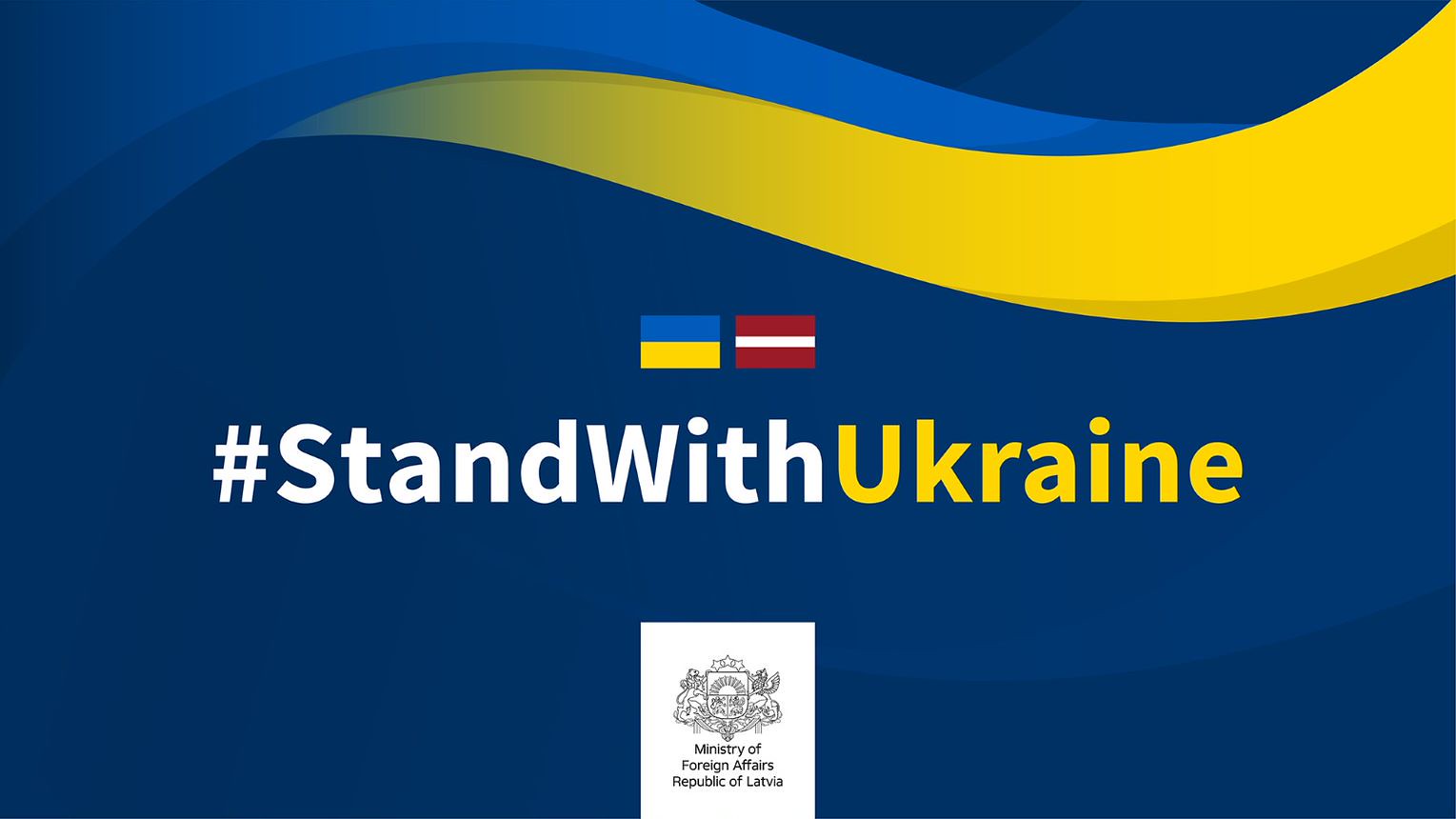The image depicts a motivational poster set against a dark blue background with a light blue and golden wavy pattern sweeping across the top. Below this design are two small flags: the blue and yellow flag of Ukraine and the red, white, and red flag of Latvia. Positioned directly in the center, the text "#StandWithUkraine" is prominently displayed, with the words "stand with" in white block letters and "Ukraine" in bold yellow. Beneath this supportive message is the emblem or coat of arms of the Ministry of Foreign Affairs of the Republic of Latvia, presented in black within a white rectangle. The overall design and colors of the poster—dark blue, light blue, golden yellow, black, white, gray, and red—underscore a message of solidarity from Latvia to Ukraine during trying times.